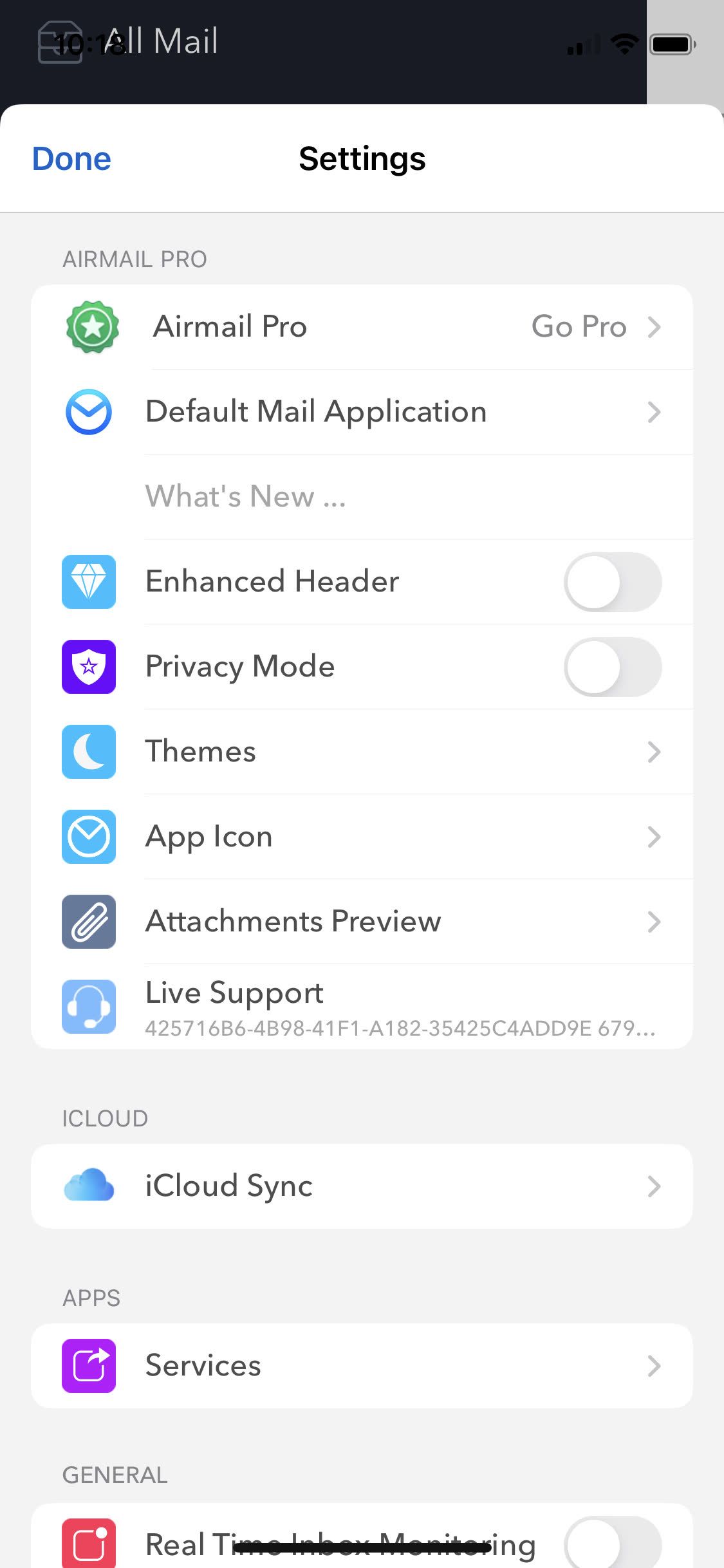Here's a cleaned-up and detailed descriptive caption for the given image:

---

The image is a detailed screenshot of a smartphone interface. At the top, a black bar displays various elements. On the left side, there is a small white logo resembling a square. To the right of the logo, in all uppercase and white font, is text that reads “AIRMAIL PRO.” At the far right, within a gray box, is a battery icon that appears full, characterized by a blacked-out center and a gray border.

Directly below the top bar, the word "Done" is prominently displayed on the left side in blue with a capital 'D.' Adjacent to it, the word "Settings" appears in black with a capital 'S,' all set against a white background in a rectangular section.

The main content area of the screenshot has a gray background and border. Inside this area, the following elements are organized in rows:

1. **Airmail PRO Section:**
   - A white-bordered rectangular area containing the text "AIRMAIL PRO."
   - Within this area, there is a green emblem featuring a white star, followed by "Airmail PRO" in capitalized letters.
   - Next to it, "GoPro" is displayed in gray with a right-pointing arrow.

2. **Blue Circle Section:**
   - A blue circle with an upside-down triangle inside it.
   - Beside this, the text "Default Mail Application" in black, with the letters D, M, and A capitalized, accompanied by a gray right-pointing arrow.

3. **What's New Section:**
   - Light gray text reading "What's New" with each word starting with a capital letter, followed by three dots.

4. **Enhancements Section:**
   - A blue box with a white diamond in the middle.
   - Text "Enhanced Header" with capital E and H, followed by a gray circular area containing a white circle.

5. **Privacy Mode Section:**
   - A purple box featuring a white coat of arms with a star in the middle.
   - Text "Privacy Mode" in gray, with capital P and M, followed by a white circle inside a gray oval.

6. **Themes Section:**
   - A white half-moon symbol inside a blue box.
   - Text "Themes" with a capital T, followed by a gray right-pointing arrow.

7. **App Icon Section:**
   - A blue box with a round symbol and upside-down arrow inside.
   - Text "App Icon" with capital A and I, followed by a gray right-pointing arrow.

8. **Attachment Preview Section:**
   - A gray box with a white paperclip icon.
   - Text "Attachments Preview" with capital A and P, followed by a gray right-pointing arrow.

9. **Live Support Section:**
   - A gray box with white headset icons.
   - Text "Live Support" with capital L and S, followed by a series of numbers and letters in gray.

10. **iCloud Section:**
    - An all-caps text "iCloud" against the gray background.
    - Below this, a white rounded rectangular area containing a blue cloud icon and the text "iCloud" with a lowercase 'i' and capital 'CLOUD.'
    - Text "Sync" in gray, with a few smaller gray dots above this section.

11. **Apps Section:**
    - Text "APPS" in gray, all caps.
    - A rectangular area with a purple square box containing a white arrow, followed by text "SERVICES" in capital letters, with a gray arrow pointing right.

12. **General Section:**
    - Text "GENERAL" in all caps and gray, beneath which is an orange square containing a white square with a dot in the right corner.
    - Text "REAL TIME MONITOR" in gray, with "REAL" and "TIME" capitalized, the latter appearing with a black line running horizontally through it.
    - Another gray circular area housing a white circle on its left side.

---

This caption comprehensively describes each element visible in the screenshot.